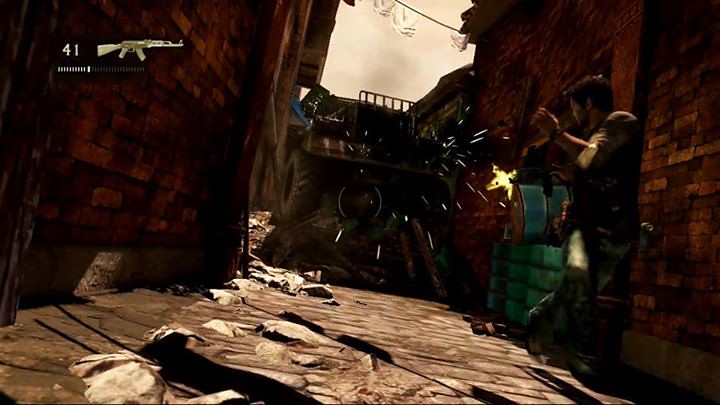This still frame from a video game depicts a narrow alleyway in an old city, characterized by its rough, multi-colored brick buildings on either side. In the upper left corner, a game HUD displays a digit '41,' a long rifle resembling a Kalashnikov, and a life bar—two-thirds depleted. The scene is vividly detailed: a cobblestone road, deformed by the advancing tank's weight, runs between the buildings. Clothes strung on a line stretch overhead, with a pink and beige garment swaying in the smoke-filled sky.

In the middle of the image, a formidable tank with large black wheels advances, spewing sparks and possibly causing explosions. To the right, a character with dark hair, dressed in a brown long-sleeve shirt and bluish pants, sprints away while looking back over his shoulder, left arm flung out and weapon firing. Yellow sparks erupt from his gun, aiming towards potential enemies clad in black in the foreground. Near him, several 55-gallon drums are stacked against the wall, suggesting recent or imminent conflict. The blend of historical and dystopian elements enhances the image's tension and urgency.